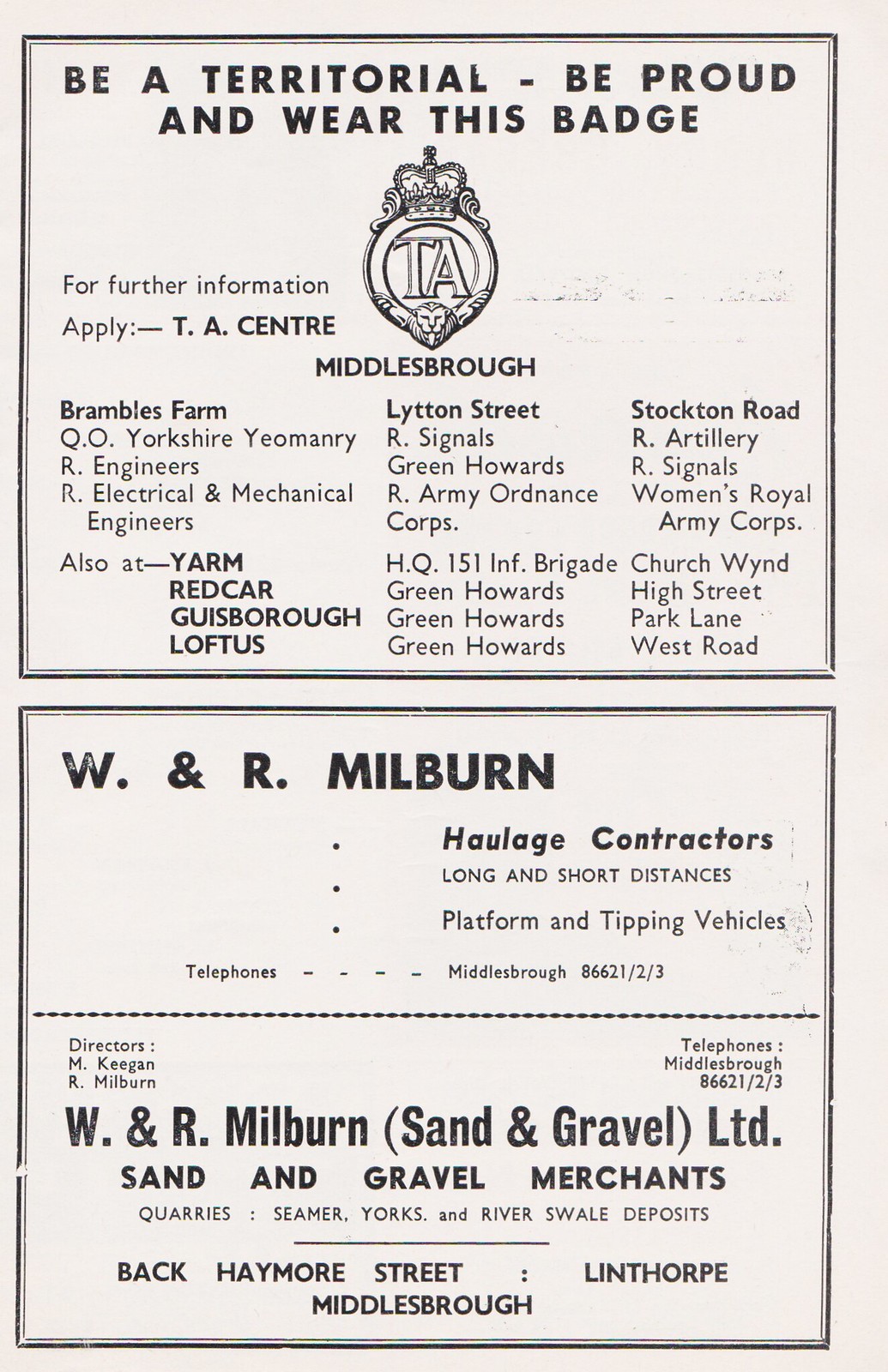This is a detailed, descriptive caption for the combined elements from the three different captions:

The image appears to be a vintage advertisement poster, predominantly white with black text and a touch of tan. At the top, in bold black letters, it reads, "Be a territorial, be proud and wear this badge." Directly beneath this phrase is an emblem featuring the initials "T.A." and the text "For further information apply T.A. Center, Middlesbrough." Below the emblem, the advertisement provides three columns listing various companies and organizations associated with different locations: Brambles Farm, Lytton Street, and Stockton Road.

The middle segment of the poster highlights "W&R Milburn, Haulage Contractors," specifying their services for long and short distances with platform and tipping vehicles. The contact information is listed as "Telephones: Middlesbrough 86621/2/3."

At the bottom of the poster, in dark print, it states "W&R Milburn, Sand & Gravel Limited," followed by "Sand & Gravel Merchants, Quarries, Seamer, Yorks, and River Swale Deposits." The address provided is "Back Hayworth Street, Linthorpe, Middlesbrough," indicating the business's location.

The detailed layout and content suggest this is an old advertisement, possibly from a phone book, with distinct sections and clear contact details, reflecting its period's typical style and design.